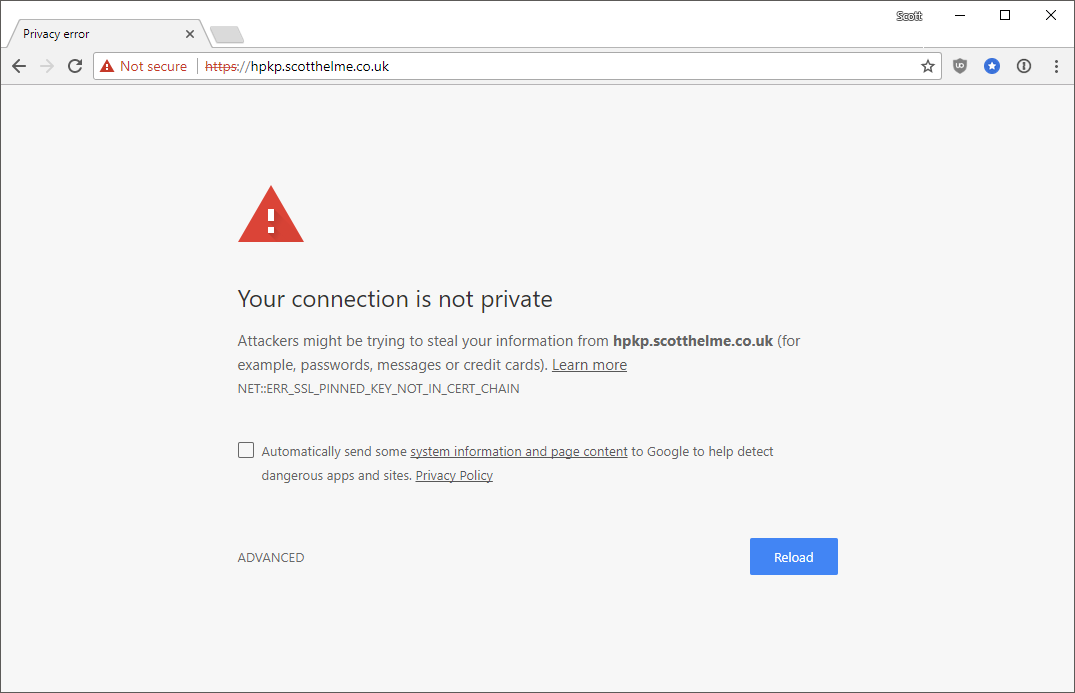The image displays a browser warning page with a prominent red triangle containing an exclamation point, indicating a security issue. The message warns, "Your connection is not private," and suggests that attackers might be attempting to steal sensitive information, such as passwords, messages, or credit card details, from the website "https://hpkp.scottholme.co.uk." The text also explains that the browser automatically sends system information and page content to Google to help detect potentially dangerous sites and applications, as per its privacy policy. Users are presented with options to "Learn more," "Advanced," and "Reload." 

At the top of the browser window, there are icons for minimizing, maximizing, and closing the window. The active tab displays "Privacy error" and notes that the site is "Not secure." Additional icons include a gray star, a shield, a blue circle with a white star, a gray circle with a diagonal line through it, and a vertical stack of three gray dots, indicating additional menu options. This intricate warning screen highlights the risks associated with continuing to the website without resolving the security issues.